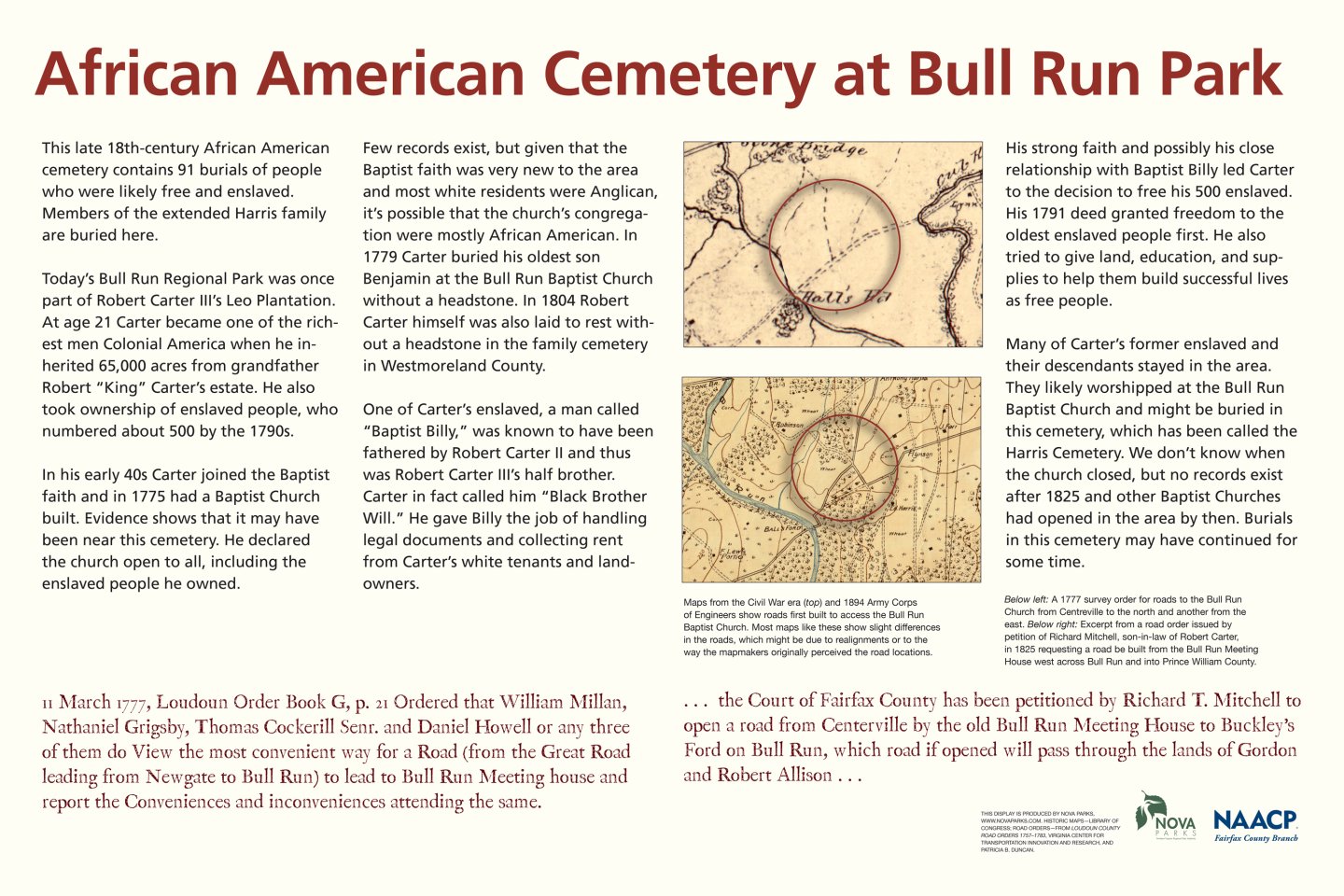The image depicts an informational sheet of paper, likely a scanned document or magazine excerpt, describing the African American Cemetery at Bull Run Park. The sheet, presented in landscape orientation, measures approximately eight and a half by eleven inches and has a yellowish off-white background. The headline, written in a large maroon font at the top, reads "African American Cemetery at Bull Run Park."

Below the headline, the document comprises around six paragraphs of small black text that detail the history and significance of the cemetery, which dates back to the late 18th century and includes 91 burials of possibly both free and enslaved African Americans. Interspersed within the text are two old-style maps, tan or beige in color, that highlight specific areas with red circles, reminiscent of centuries-old cartography.

At the bottom of the document, there are two paragraphs in small maroon font that describe an event from 1777 related to the cemetery’s history. Positioned in the lower right corner are two logos: one for the NAACP and another labeled "NOVA," situated just to the left of the NAACP logo. The overall layout and historical maps aim to inform visitors about the cemetery's background and its significance within Bull Run Regional Park, which was originally part of Robert Carter's plantation.